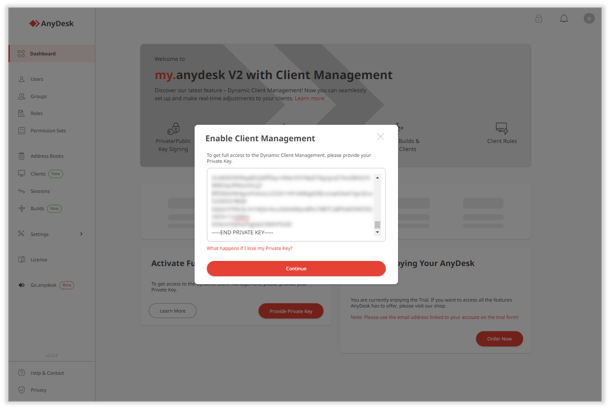This image depicts a webpage from the company AnyDesk. In the upper left corner, the AnyDesk logo is displayed in black, accompanied by an icon featuring two diamond-shaped boxes, one positioned behind the other. The page title reads "My Any Desk v2 with Client Management," and the overall color scheme is predominantly gray.

Central to the webpage is a prominent pop-up message that states "Enable Client Management." It appears to provide instructions for enabling this feature, although the text within the pop-up box is intentionally blurred, rendering the details unreadable. At the bottom of this pop-up, there is a large red button labeled "Continue."

The main section of the webpage features a partially visible message in bold black letters that reads "Activate," followed by obscured text about "carrying your AnyDesk." The gray background makes this text difficult to decipher.

On the left side of the page, there is a vertical dashboard with various categories listed, providing navigational options for users to explore as needed. The overall design conveys a detailed and complex interface tailored for client management within the AnyDesk platform.